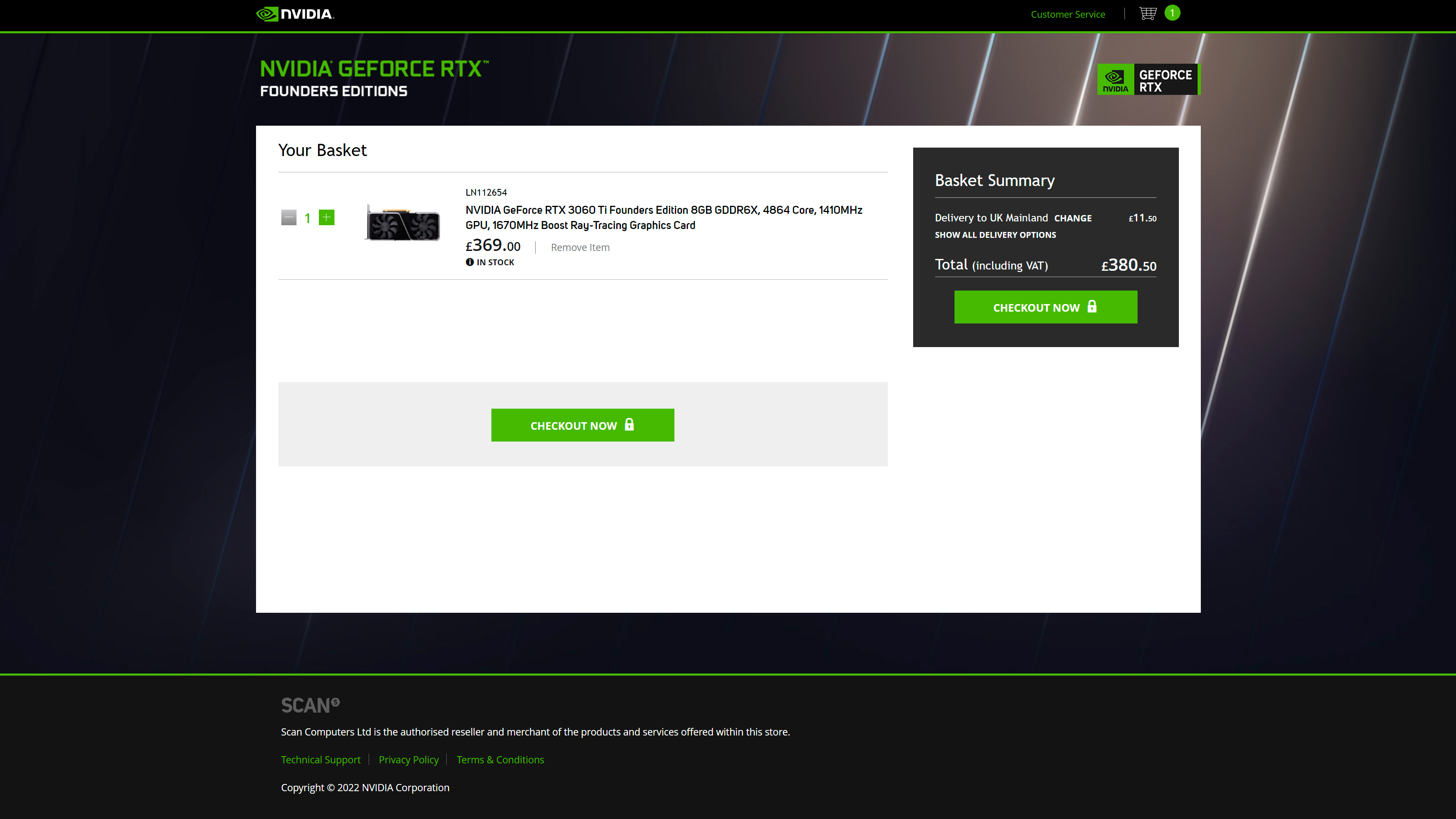The image depicts a landscape-oriented, rectangular webpage for a technology-based company, likely NVIDIA. At the top of the page, there is a thin green horizontal line separating the black border above it from the rest of the content. Within this black border, the white NVIDIA logo appears on the left-center, accompanied by a green logo. To the right of the logo, there are icons for customer support, a shopping cart, and a green circle.

Beneath this header, the webpage has a black background adorned with diagonal white lines. Prominently displayed is the text "NVIDIA GeForce RTX" in green, with "Founders Edition" written in white underneath. Further down, another NVIDIA logo and the text "GeForce RTX" appear within a dual-colored green and black box.

Below this section is a white, rectangular box labeled "Your Basket." Inside this box, there is a picture of the NVIDIA GeForce RTX item alongside its specifications, which are difficult to read. The item is listed for sale at a price of 369 units of an unspecified foreign currency. A green, rectangular "Checkout Now" button with white font is positioned below.

To the left of this shopping summary is a detailed "Basket Summary," which includes a delivery charge of 11 units of the currency and a total cost of 380 units. Another green, rectangular "Checkout Now" button is located here as well.